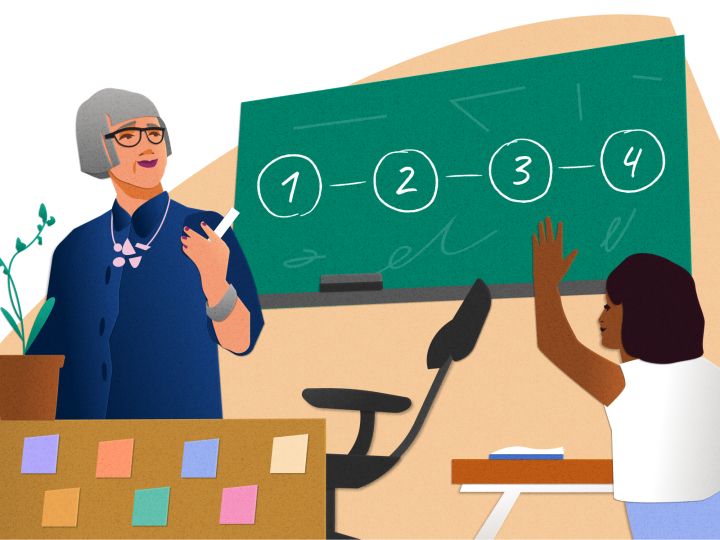The image depicts a detailed digital illustration with a high contrast of colors. Set against a white and peach background, the foreground features a white-skinned teacher with short gray hair and glasses, standing beside her desk. In her right hand, she holds a piece of chalk and appears to be engaging with an African American student seated at a nearby desk with her hand raised, seemingly ready to answer a question. The teacher is dressed in a blue dress, adorned with a pink-accented necklace, and a gray watch, with her nails painted. Her desk is cluttered with colorful post-it notes and a green plant, while a black office chair is parked behind it. Dominating the upper section of the background is a green chalkboard which displays four numbered circles, 1 through 4, connected by dashes. The student, dressed in a white shirt and blue bottoms, attentively gazes at the teacher, creating an interactive and vibrant classroom scene.